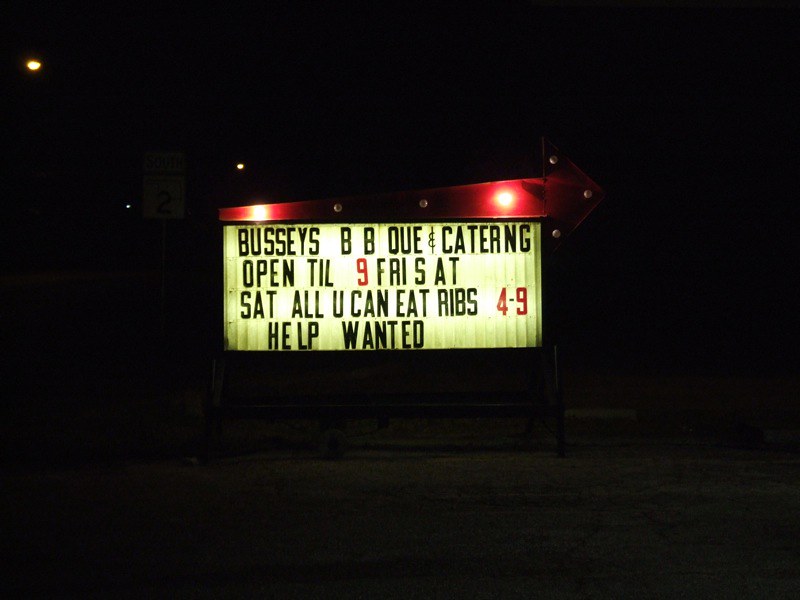In this nighttime photograph of a rectangular restaurant advertisement sign, the scene is predominantly dark, illuminated by a few bright, yellowish lights in the top left corner, likely from distant streetlights. The main focus of the image is a billboard-style sign with a red top border and a yellow backlit background that enhances its visibility. The sign features black text and some red numbers, reading: "Bussy's BBQ and Catering, open till 9, Fri, Sat, Sat, all U can eat ribs, 4-9, help wanted." The sign appears handcrafted, typical for customizable outdoor displays. The surrounding area is obscured by darkness, with no other details visible except for the faint illumination from the aforementioned lights.